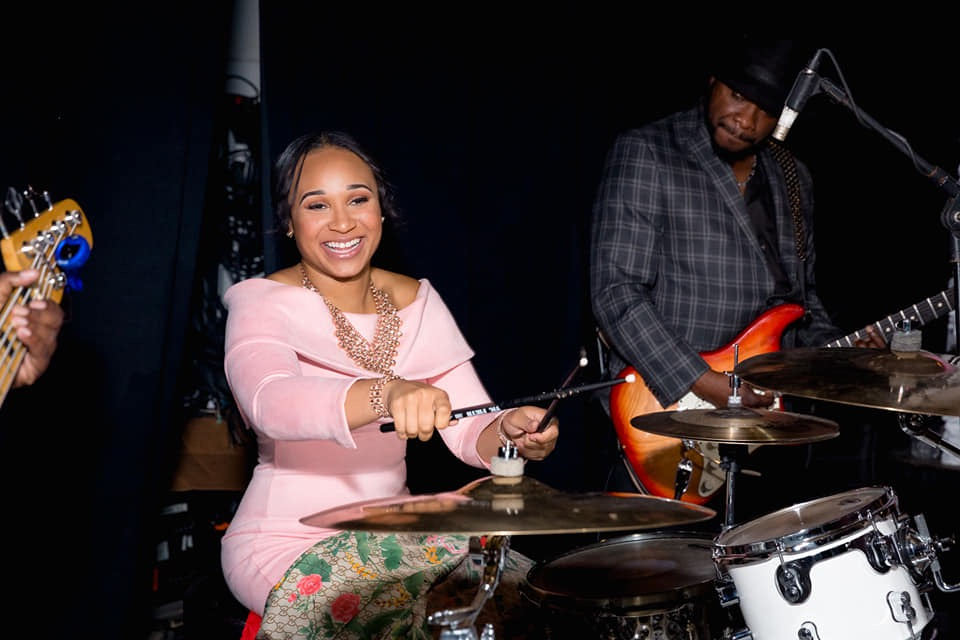In the image, a band is performing against a dark backdrop, possibly a stage area with a dark blue curtain that has a partially open slit revealing an off-stage area. Central to the scene is a female drummer and a male guitarist. The drummer, a woman in an elegant pink dress with a floral pattern, is adorned with a chunky gold necklace and a matching bracelet. She is smiling brightly, exuding happiness, while holding black drumsticks crossed over each other. In front of her are white drums and bronze-colored cymbals. To her left is a male guitarist, dressed in a black and gray checked suit jacket over a black t-shirt, and wearing a black hat. He is playing an electric guitar that is predominantly red with a hint of yellow highlight. Positioned above him is a microphone. To the far left edge of the image, the hand of another musician, possibly a bassist, is visible holding the light brown head of their instrument. The guitarist is turned slightly towards the drummer, seemingly looking at her while they perform.